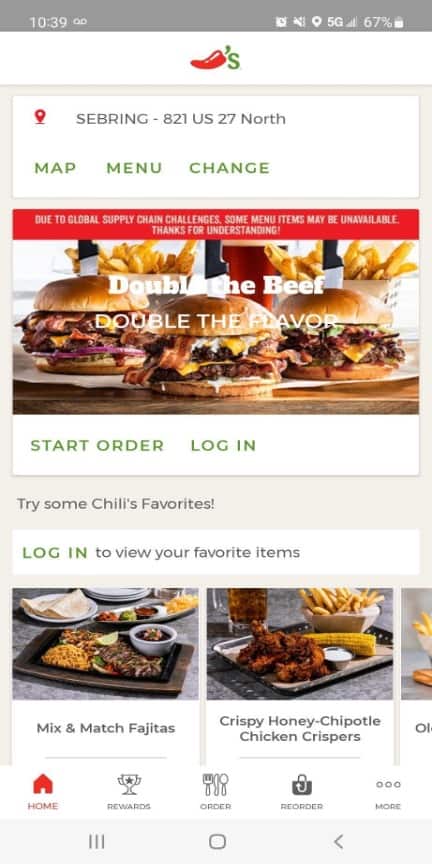This image is a screenshot of a Chili's menu interface on a mobile phone, meticulously detailing various features and items on the screen. At the very top, a gray status bar displays the time as 10:39, flanked by seven icons indicating the phone's status: location, 5G connectivity, signal strength, and battery level, which is at 67%, all in clean white font.

Directly beneath this, the iconic Chili's logo is prominently displayed, featuring a red chili pepper with an apostrophe and 'S' in green. Below the logo, a white search box specifies the restaurant location with a red location marker and the address "Sebring-821US27N." Adjacent to this, three navigation options are presented in green: Map, Menu, and Change.

A large, appetizing photograph showcasing three double beef sandwiches on fresh rolls, accompanied by French fries, dominates the central area of the screen. The image is overlaid with the text "Double the Beef, Double the Flavor," enticing the viewer with a promise of hearty satisfaction.

Below the photograph, a white bar offers the options "Start Order" or "Log In" in vibrant green font, prompting user interaction. Following this, a promotional section invites users to "Try Some Chili's Favorites" with an added message to log in to view personalized favorite items. 

The screen further showcases two visually appealing platters set against a gray table backdrop. One platter is laden with sizzling side fajitas, Spanish rice, and a bowl of black beans, while the other presents crispy honey chipotle chicken crispers, accompanied by an ear of corn, French fries, and a refreshing iced tea.

Finally, at the bottom of the screen, five intuitive icons guide user navigation: a red house for the home screen, a trophy for rewards, a knife and fork for ordering, a bag with an arrow for reordering, and a 'more' option, ensuring a comprehensive user experience.